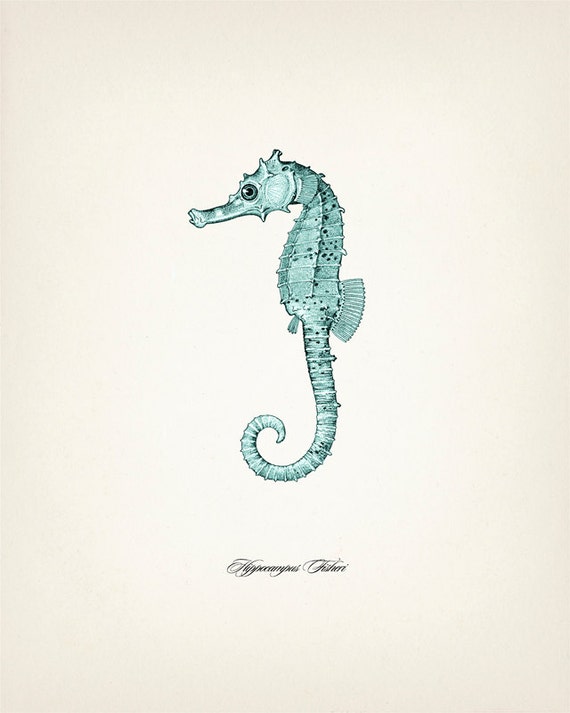This detailed drawing showcases a young seahorse prominently centered on a beige paper background. The seahorse, rendered in intricate detail, appears primarily in a light greenish-teal hue with interspersed bits of white and black spots. The texture clearly shows the segmentation of its tail and body, with every small line meticulously drawn. Its large black eye with a gray iris and a prominent snout are distinctive features. The tail curls into a spiral, with a flared fin around its hindquarters. Below the seahorse, in fine cursive script, is its Latin name, starting with "hippocampus" though the second word is indecipherable. The seahorse’s delicate fins and other features are vividly brought to life, giving it a sense of movement as it seems to look off to the left of the image.